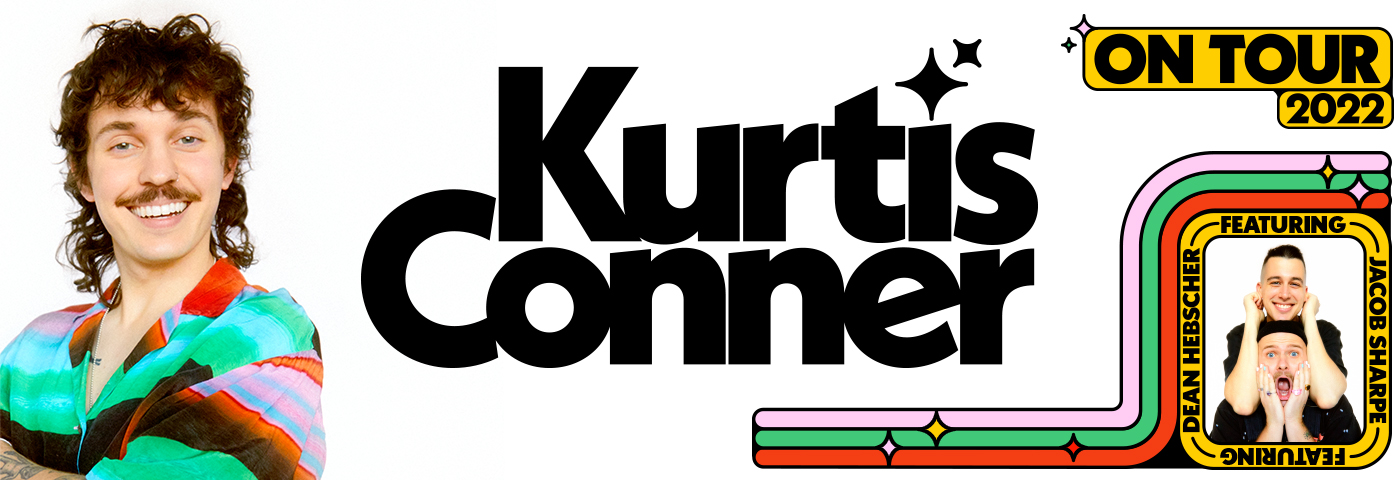The image is a vibrant, 1980s-style advertising poster or ticket back for an entertainment tour, likely comedy. On the far left, there is a photograph of a medium to light-skinned man with long, dark, curly hair and a mustache, smiling widely. He is wearing a striped shirt that features colors like red, green, black, turquoise, and blue. Large black letters in the middle of the poster spell out "Curtis with a K Conner," with the dot on the 'i' replaced by a star and another star floating nearby. In the upper right-hand corner, in bold black text on a yellow background, it reads "On Tour 2022." Adjacent to this, there is a banner with three lines in pink, red, and green, which match the colors of Curtis's shirt. Below, there is a box enclosing photographs of two men; the man on top is holding his earlobes, while the man below has his hands behind his ears. Text around the box states "Featuring Dean Hebscher and Jacob Sharp." This detailed and colorful poster clearly promotes Curtis Conner and his tour for the year 2022, highlighting additional performers Dean Hebscher and Jacob Sharp.